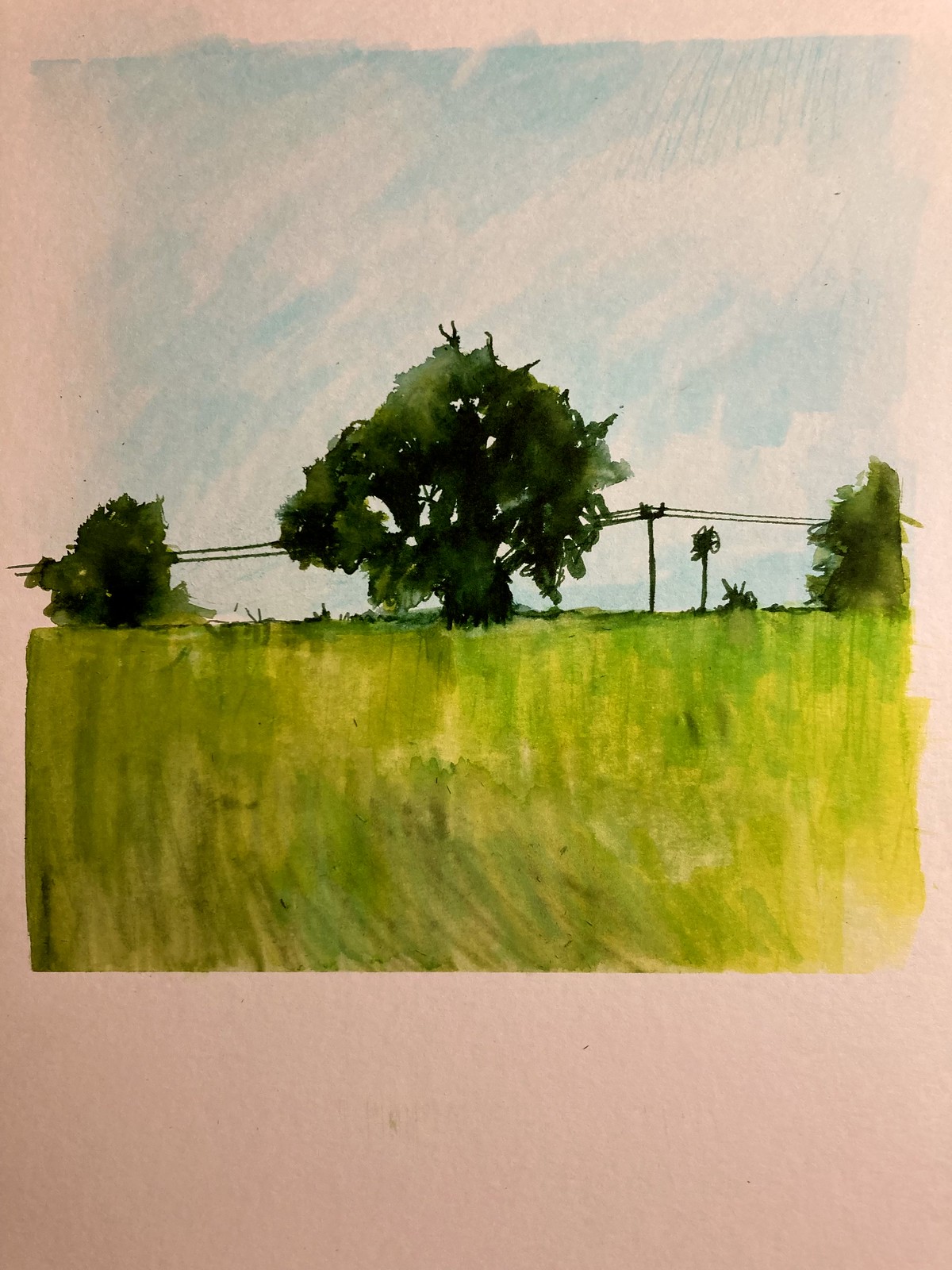This is a watercolor-like painting on pale pink paper, depicting a serene landscape. The foreground features a grassy meadow shaded with light kelly green and yellow markers, extending up to the bottom quarter of the image where it abruptly transitions into the pink background. Dominating the scene is a large, leafy tree centrally positioned, flanked by two smaller trees on either side. In the background, power lines stretch horizontally between the trees, adding a touch of rustic charm. The sky above is rendered in a soft, airy blue that allows the pink of the paper to peek through, and it's dotted with whimsical pink and white clouds, creating a dreamy atmosphere. The overall composition is light and delicate, blending the pastel hues with darker accents for a balanced, calming effect.